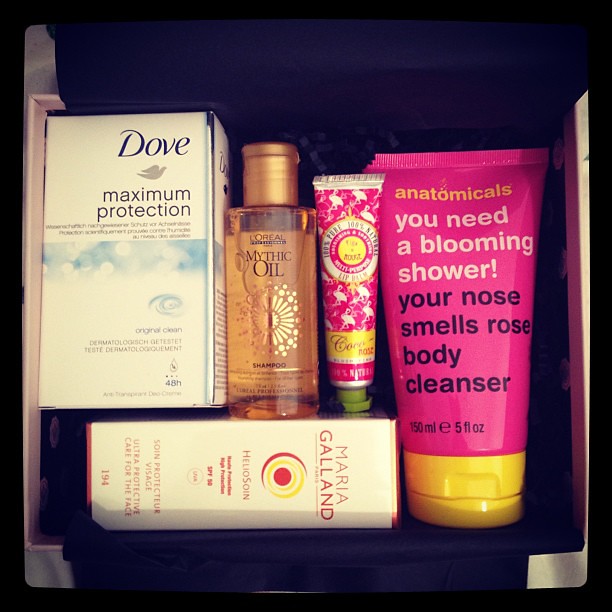The photograph features a collection of bath and body products neatly arranged inside a white box with navy blue lining, which has a circular pattern, possibly floral. The items include a white box labeled "Dove Maximum Protection" with blue lettering. Adjacent to this is a small, clear bottle of L'Oreal Mythic Oil shampoo, featuring a gold cap and a gold starburst design. Following that is a small, colorful tube of lip balm, decorated in pink, white, and yellow, with a green tip and a white flamingo pattern accompanied by a yellow band. Further to the right is a prominent fuchsia tube with yellow accents, labeled "anatomicals. You need a blooming shower. Your nose smells rose. Body cleanser," with a yellow cap. Lying horizontally at the bottom of the box is a small, rectangular white box that reads "Maria Galland. Heliosign. Ultra protective care for the face," which includes SPF, indicating it is a type of sunscreen.